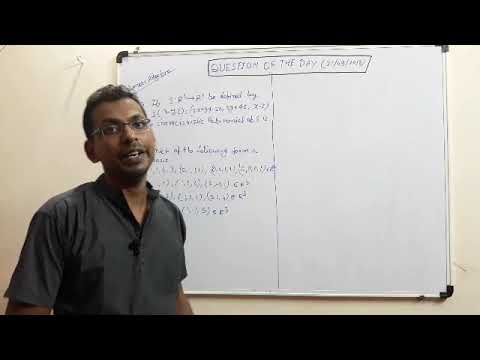This color photograph captures a young man, likely in his early 30s and of Indian or Middle Eastern descent, standing on the left side of the frame. He has short, dark, curly hair, is slightly balding, and sports glasses along with a mustache and goatee. He's wearing a black collared shirt with a microphone clipped to it, and appears to be in mid-sentence, suggesting he's delivering an instructional lecture, possibly related to math. Behind him is a whiteboard attached to a beige-colored wall, divided by dotted lines down the middle. At the top of the board, the phrase "Question of the Day" is written prominently in marker. The whiteboard is filled with black and blue writing, and although some of the text is fuzzy and largely unreadable, it features a series of mathematical equations. The image is framed with black bands above and below, adding a cinematic quality to the scene.